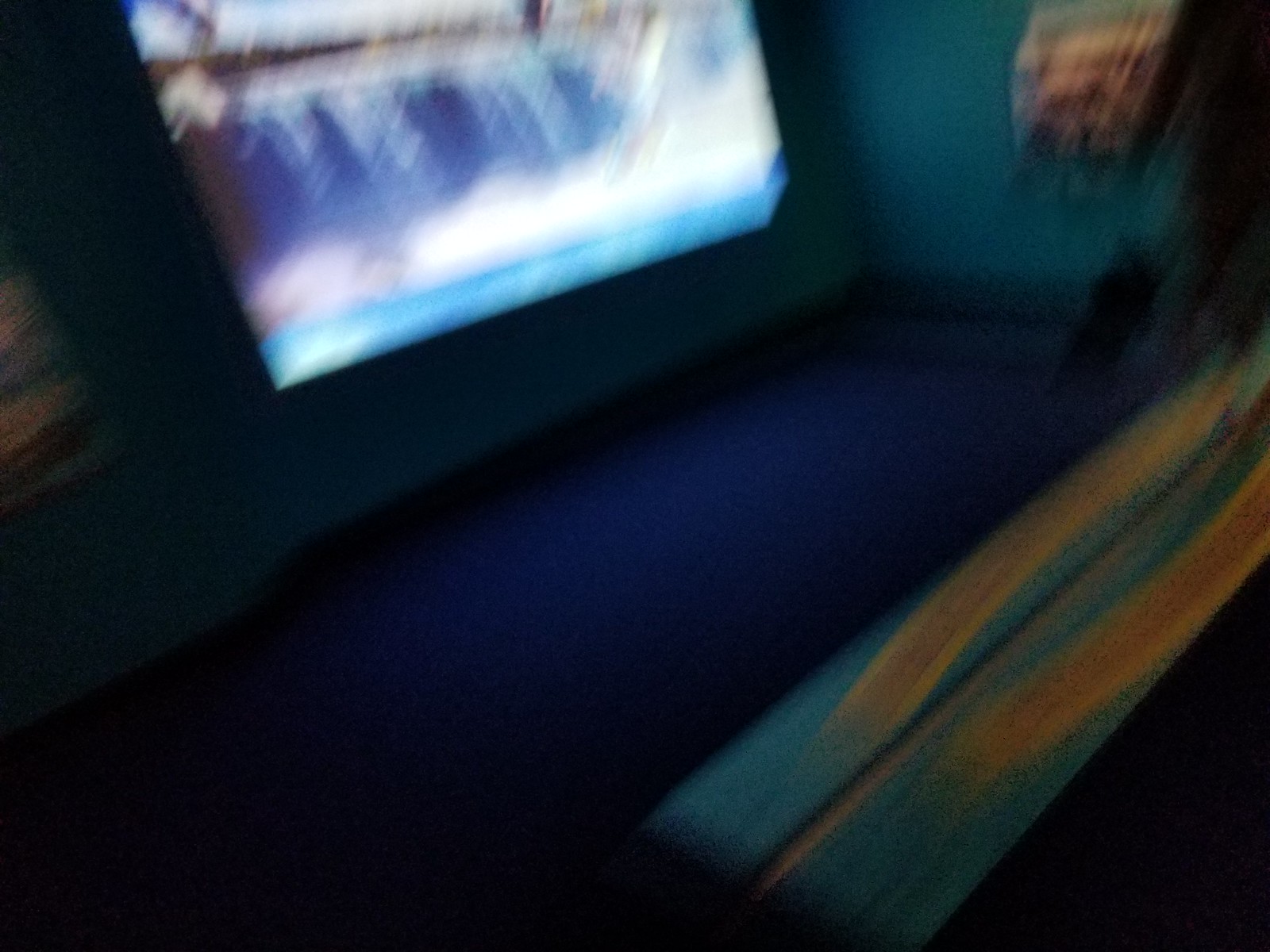In this blurry, nighttime photograph dominated by shades of blue, the upper left-hand corner features a bright rectangle emitting white and blue light, possibly resembling a TV screen. Adjacent to this, a patch of dark greenish-blue is accented by brown and black hues in the upper right-hand corner. The lower right-hand section of the image displays two elongated streaks of dark blue-green, topped with lighter brown, creating a contrast against the surrounding darkness. The composition appears abstract, with distinct but obscured shapes and colors contributing to its enigmatic quality.